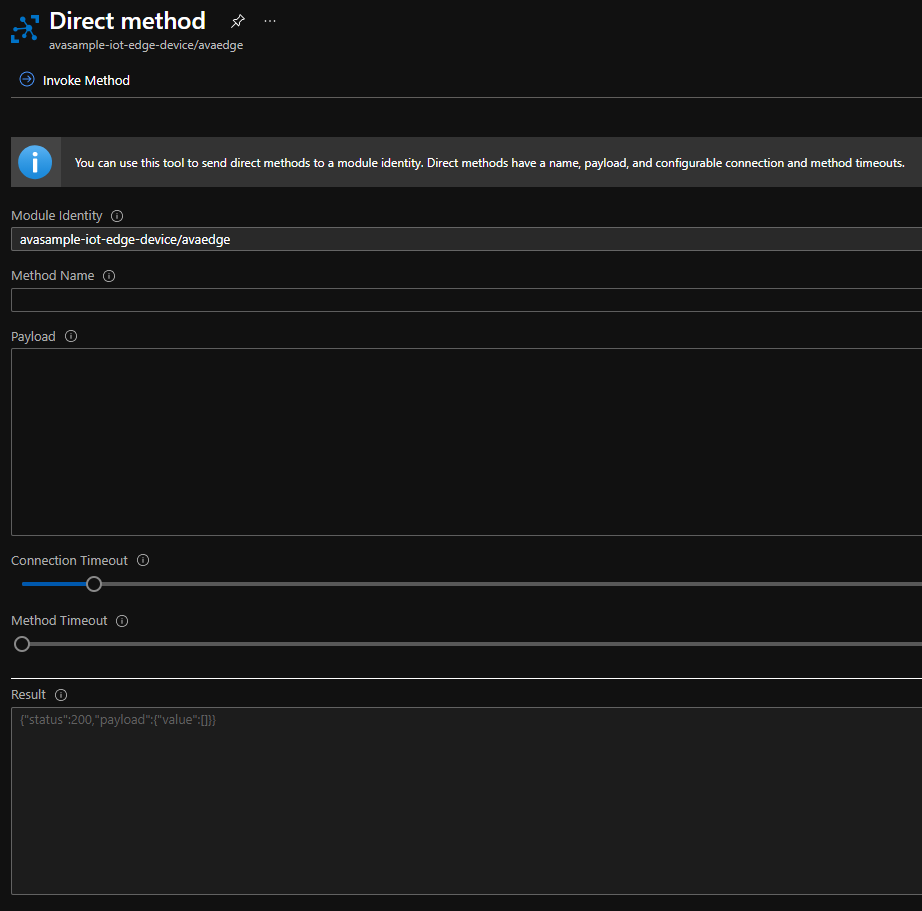**Caption:**

The screenshot features a web page dedicated to the "Direct Method" functionality. At the top, the title "Direct Method" is prominently displayed, followed by "ava-sample-IOT-edge-device/AVA-edge." To the left of the title is a distinctive blue logo made up of dots interconnected with lines, featuring an arrow pointing down-left and another pointing up-right. Adjacent to the title is a pin icon and a button with three horizontal dots, indicating additional options.

Below the main title, there is a subsection labeled "Invoke Method." This is followed by an informational bar that explains the tool's purpose: "You can use this tool to send direct messages to a module identity. Direct methods have a name, payload, and configurable connection and method timeouts." Accompanying this text is a blue icon featuring a white "i" for information.

Further down, user-interactive fields are presented. The first field, "Module Identity," is pre-filled with the text "ava-sample-IOT-edge-device/AVA-edge." The "Method Name" and "Payload" fields are blank, awaiting user input. Below, there are two sliders: the "Connection Timeout" slider is slightly moved to about 10-15% of its full range, while the "Method Timeout" slider remains untouched at the far left. The final field, "Result," is pre-populated with placeholder text that reads "status: 200, payload: {}, indicating no current result data.